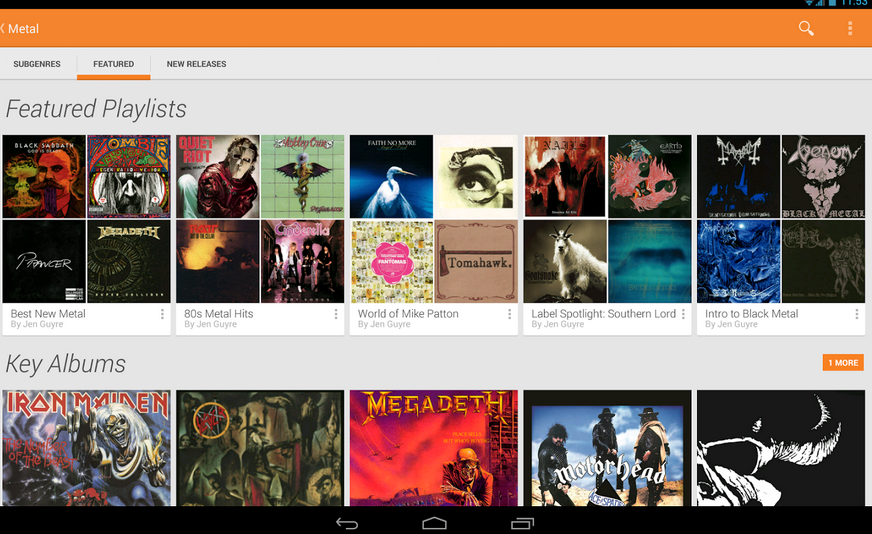In this screenshot of a music app, detailed elements are neatly captured. At the very top right, partially cut off, the time reads 11:53, accompanied by full WiFi signal bars, and a phone signal icon showing nearly full strength (about three or four bars). On the top left, the word "Metal" in white text is visible next to an "X" icon, with a magnifying glass and three-dot icon located to the far right. This top section is set against an orange background.

Below the header, there are three navigational categories: "Subgenres" on the left, "Featured" in the center with an orange rectangular highlight bar underneath, and "New Releases" on the right.

The main section displays "Featured Playlists" with a grid of album covers. There are four album covers per square, arranged in five squares. From left to right, the first square is labeled "Best New Metal," the second "80s Metal Hits," the third, positioned centrally, is "World of Mike Patton," the fourth is "Label Spotlight: Southern Lord," and the fifth square is "Intro to Black Metal." Each square showcases assorted album artworks, offering a visually engaging overview of various metal music playlists.